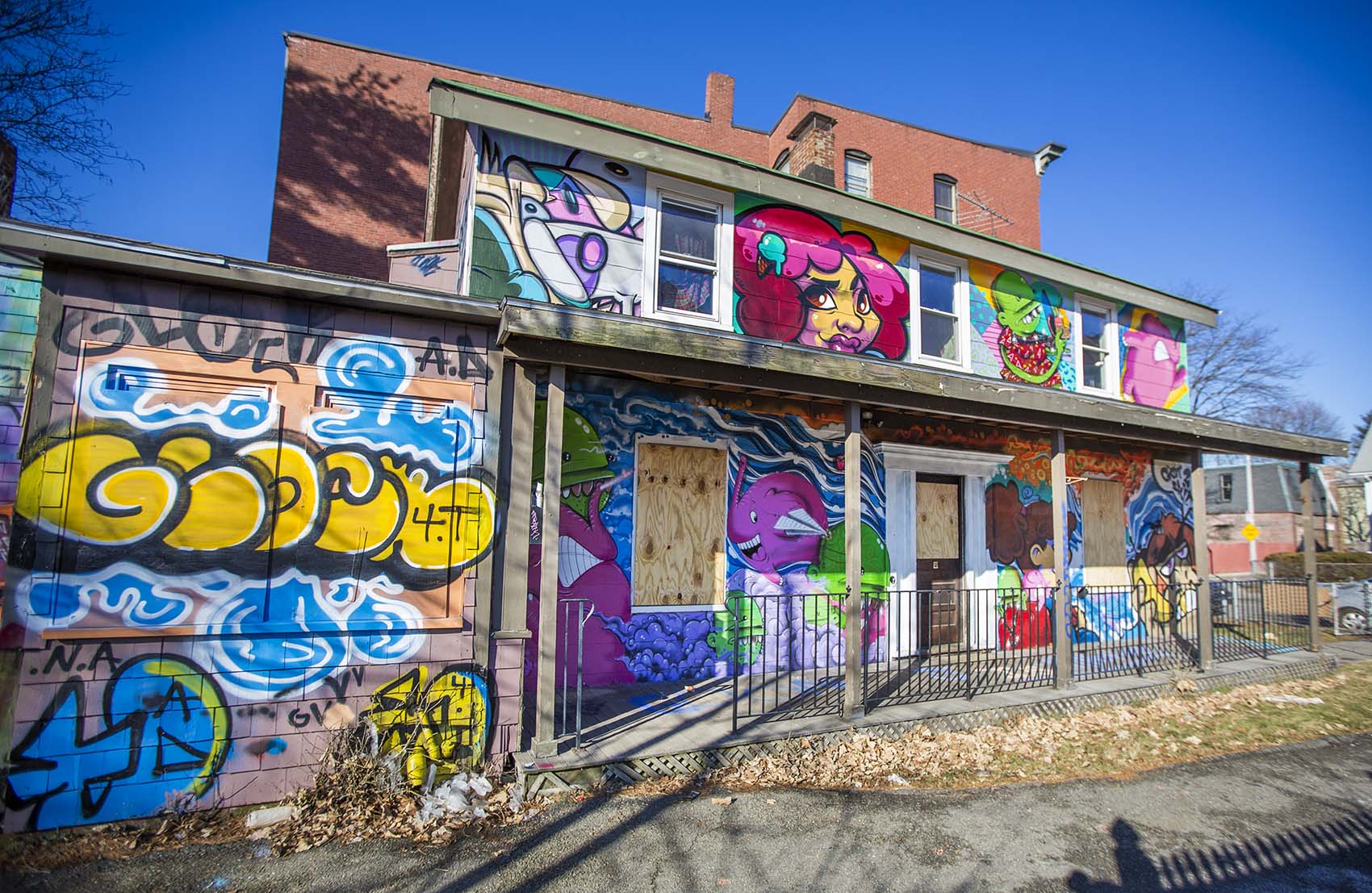The photograph captures a dilapidated and abandoned two-story house under a clear blue sky. The building’s ground floor windows and doors have been boarded up with wooden planks, leaving no glass visible. The exterior of the house is extensively decorated with vibrant graffiti in various colors and styles, including images of a cartoonish female character with bright pink hair, a green monster, a large, smiling purple elephant, and several other colorful figures. Additionally, there are cartoon-like shapes and letters, notably a partially legible name or phrase with blue figures beneath, possibly "N.A."

A front porch connects the building to the sidewalk with a metal railing and light pine-colored vertical posts supporting the overhang of the roof. The brown front door, featuring a glass pane at its top, is framed by a white square archway. Scattered brown leaves cover the concrete area in front of the porch, blending into a small, disordered half-circle patch of grass. In the background, a large red brick building looms behind the house, with additional buildings and the edges of several vehicles slightly visible to the far right. Shadows of an unseen fence fall at the bottom right corner of the image, further accentuating the isolated and neglected nature of the scene.